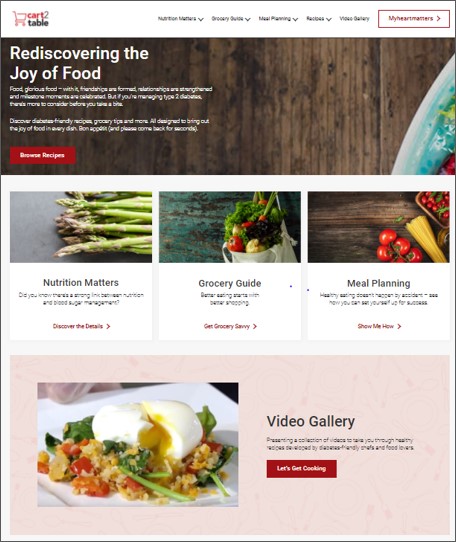Screenshot of a webpage from a meal and nutrition planning service. At the top left is a small shopping cart icon with the text "Cart 2 Table." The navigation menu runs across the top, with partially legible options such as "Meals," "Nutrition," "Grocery Guide," "Meal Planning," and "Recipes." One option, blurred but distinguishable in red, reads "My Heart."

Below the menu, a large banner with a logo featuring the edge of a plate is overlaid with the text "Rediscovering the Joy of Food." Following this, there are two white paragraphs of text, which are difficult to read in detail. Directly beneath this text is a prominent red button labeled "Browse Recipes."

Further down, the page displays three images aligned horizontally across the screen. The left image depicts asparagus and is captioned "Nutrition Matters." The center image shows a grocery bag filled with fruits or vegetables, with the caption "Grocery Guide." The right image features tomatoes and peppers, tagged with "Meal Planning."

At the very bottom of the page, a pink rectangular section spans the width of the screen. It includes a picture of a meal and the label "Video Gallery."